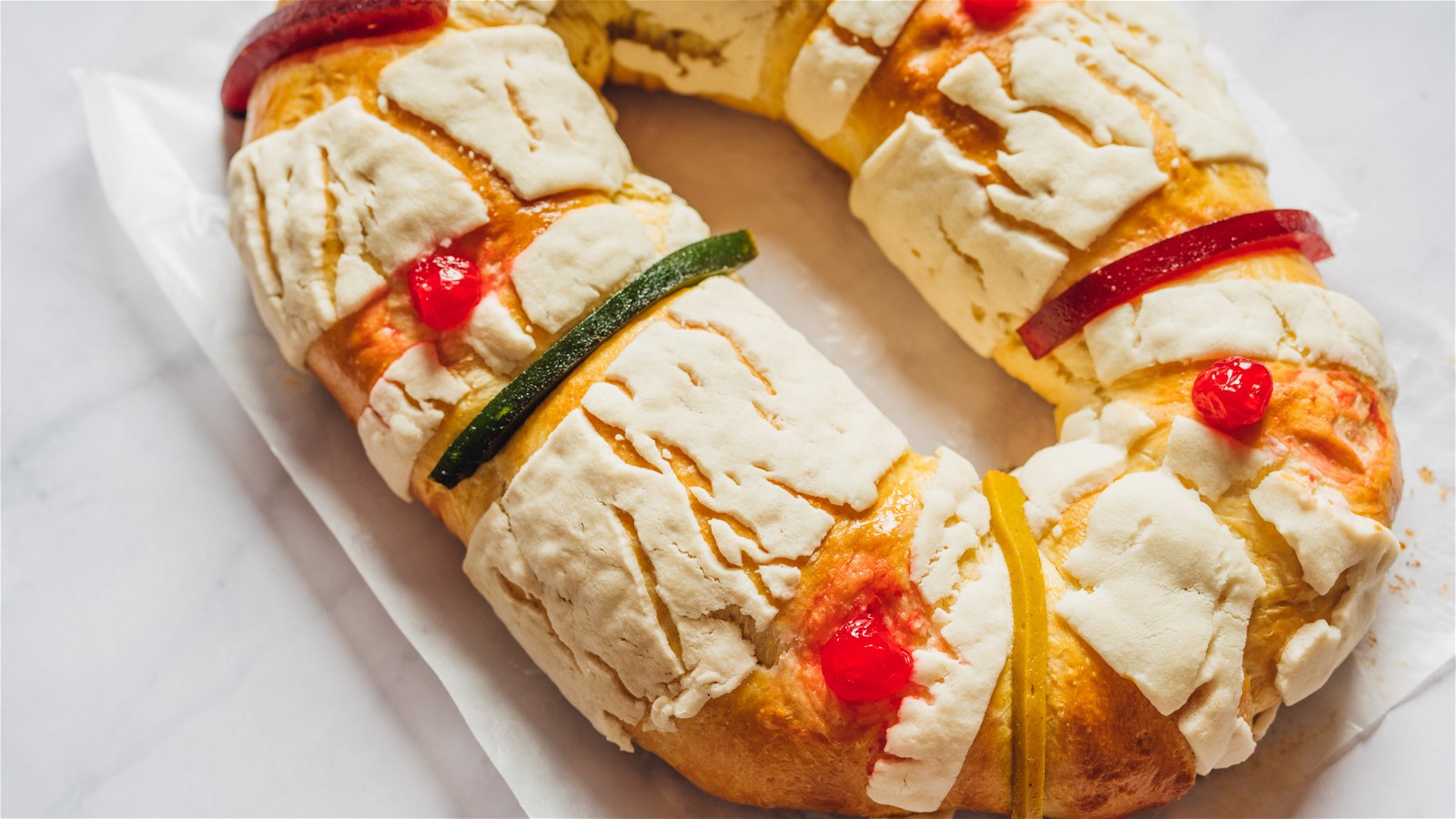The landscape-oriented photograph captures a uniquely shaped pastry that resembles an oblong doughnut or oval with two pronounced areas of thickness on the sides connected by a loop at the bottom. It rests on a piece of white parchment paper that fits the bread perfectly, which in turn is placed on a white and light gray marble countertop. The pastry is decorated with a variety of colorful toppings: a combination of melted white cheese and possibly icing, creating a base layer. On top of this, there are visible strips of red, green, and yellow bell peppers or candies, arranged in a repetitive pattern around the bread. Additionally, dried tomatoes and maraschino cherry-like toppings are sprinkled across the surface, adding to its decorative appeal. This detailed arrangement suggests a blend of savory and sweet elements, making the bread both visually striking and intriguing.